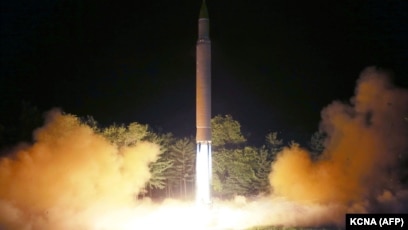The night sky serves as a dramatic backdrop in this real-life photograph of a rocket launch. Centered in the image is a long, slender rocket with a smooth, cylindrical body and a darker tip, devoid of any identifying marks or appendages. The rocket, mostly white in color, is being propelled upwards by a brilliant, white-hot explosion of fuel at its base. This fierce propulsion creates a plume of glowing smoke that billows out to the left and right, transitioning in color from bright orange and yellow near its source to deeper reds and blacks as it dissipates. In the illuminated background, a line of trees stands visible, bathed in the fiery glow of the rocket's launch. The bottom right-hand corner of the photo features a watermark saying "KCNA AFP," subtly marking the image's source.